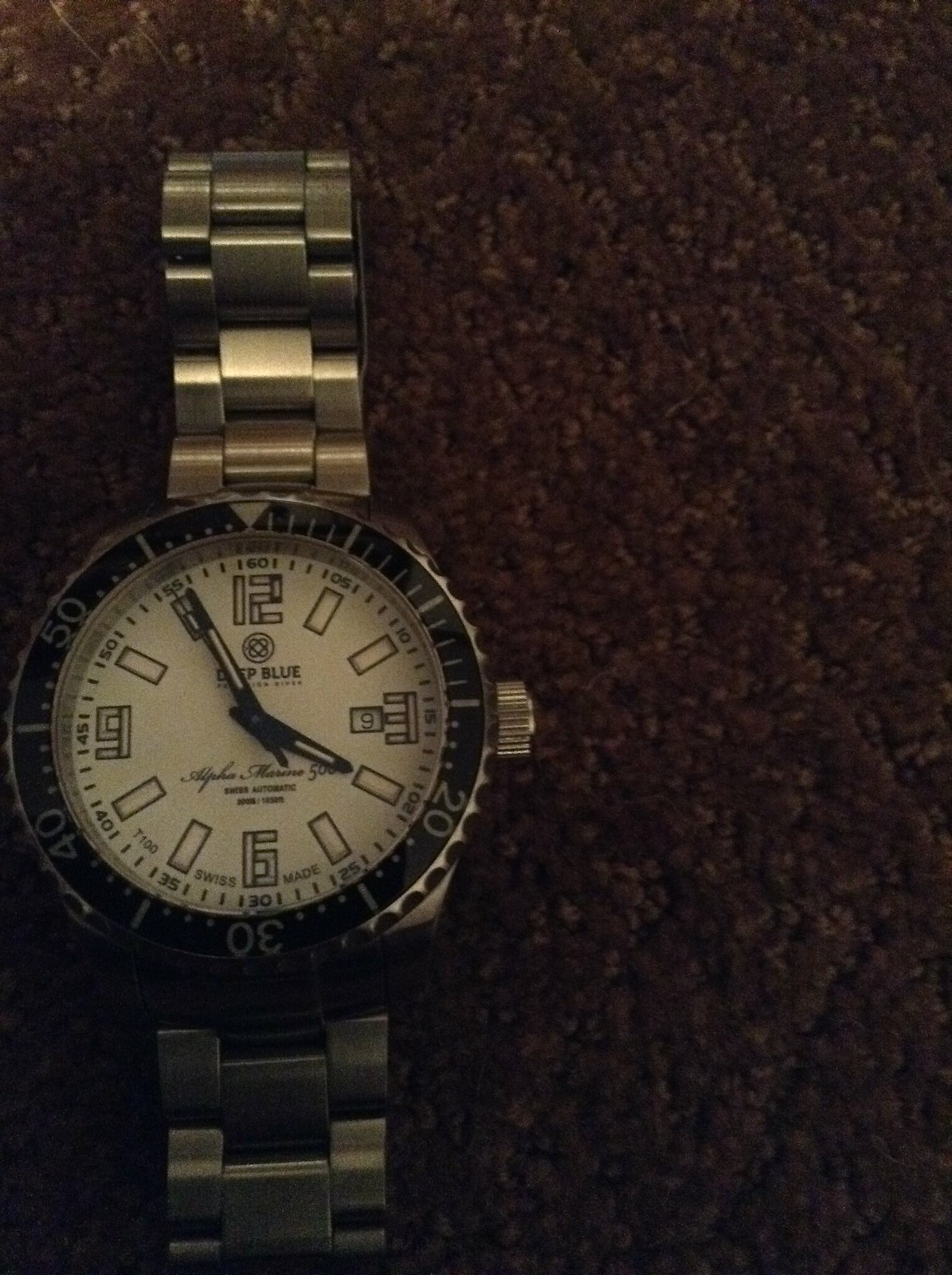A close-up image features a wristwatch positioned towards the left side against a dark red background. The watch has a circular face with a silver knob located on the right side. The watch band is also silver, complementing the knob. Encircling the watch face is a black bezel marked with numerical indicators at intervals, reading "20, 30, 40, 50" in a counterclockwise direction starting from the bottom right. The inner dial of the watch is white, providing a striking contrast to the black bezel.